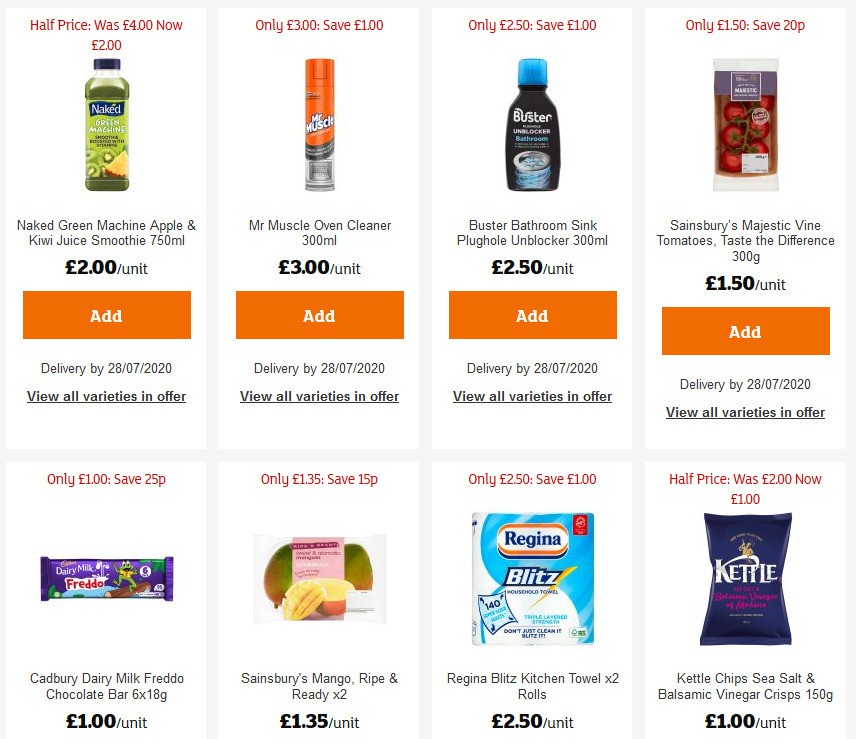An online grocery website showcases an assortment of eight different products. 

At the top left, there is a 750ml Naked Juice Drink, specifically the Green Machine Apple and Kiwi Juice Smoothie, priced at £2 per unit. Currently, it is on a half-price sale. Beneath it, an orange button invites users to add it to their cart, with an expected delivery date by 28-07-2020. There is also a link provided to explore all available varieties on offer.

Next is the Mr. Muscle Oven Cleaner, available in a 300ml bottle for £3 per unit. Following that, there is the Buster Bathroom Sink Plug Unblocker, also 300ml, priced at £2.50 per unit.

In the fresh produce section, Sainsbury's Majestic Fine Tomatoes, under the "Taste the Difference" range, are displayed in a 300g pack for £1.50 per unit.

In the confectionery section, there's a Cadbury Dairy Milk Freddo Chocolate Bar priced at £1 per unit.

The fruit section includes Sainsbury's Mangoes, Ripe and Ready, in a pack of two for £1.35 per unit.

The household essentials feature the Regina Blitz Kitchen Towel, available in a pack of 2 rolls for £2.50 per unit.

Lastly, there are the Kettle Chips Sea Salt and Balsamic Vinegar Crisps, priced at £1 per unit.